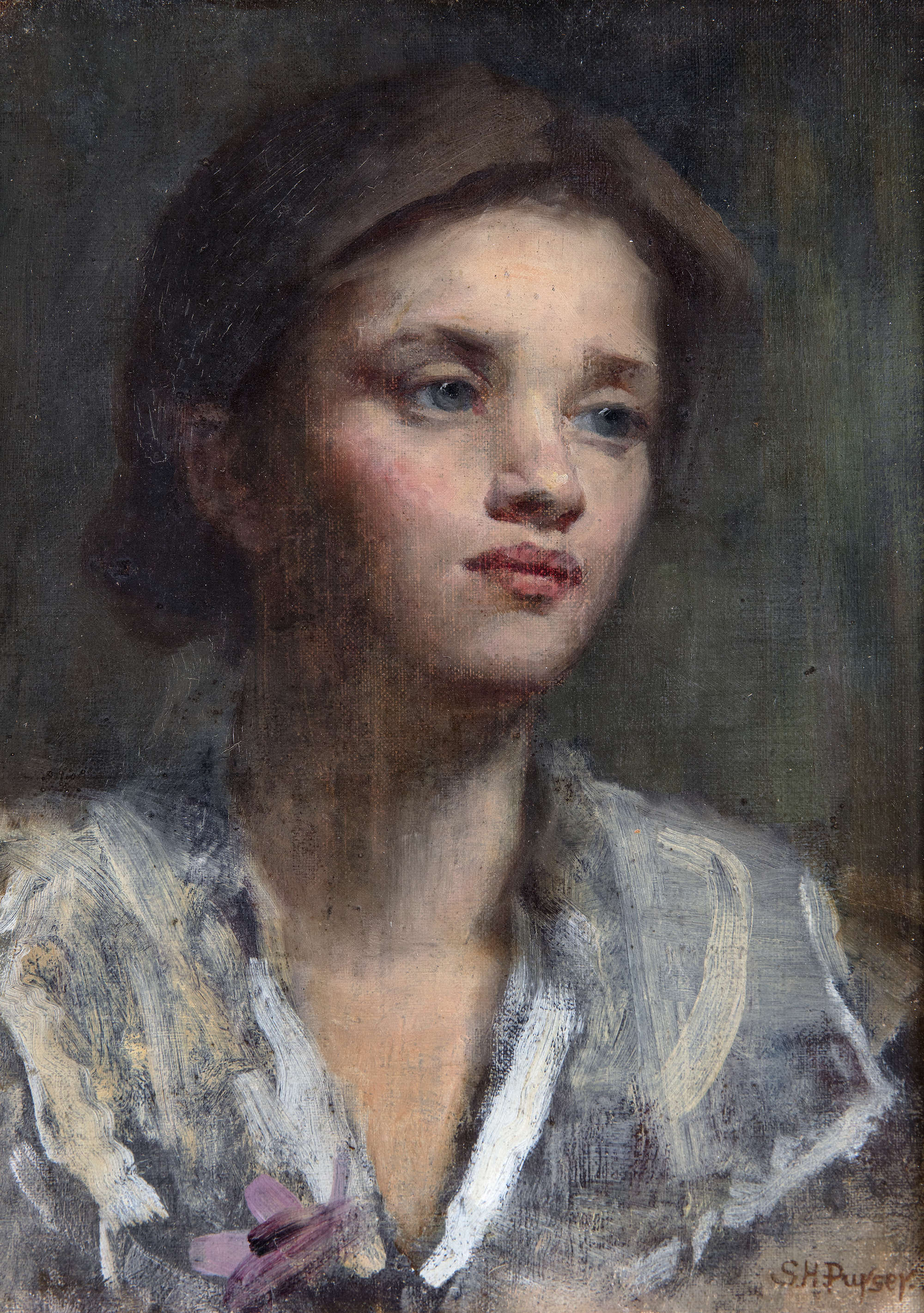This rectangular painting, oriented vertically, depicts a young woman from the chest upwards. She has light-colored skin, bright blue eyes, red lips, and brown hair styled in a low bun at the back of her neck. Her face, positioned nearly center but slightly towards the top, displays a thoughtful or slightly bored expression, with shadowing on the left side. She wears a grayish-blue dress with a v-neckline and a reddish-pink flower pinned to the left side of her chest. The background consists of dark gray and black tones. Notable is the signature of the artist, "S-H-P-U-Y-S-E-Y," visible in the bottom right corner. The detailed and carefully rendered face contrasts with the smudged depiction of her dress, adding an intriguing texture to the artwork.